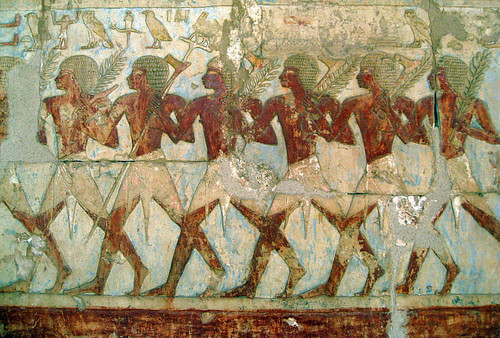The image depicts a highly distressed and decayed ancient Egyptian wall painting characterized by significant cracks and mold. The mural features seven dark-skinned men, each wearing white linen skirts that extend to their knees, rendering them bare-chested. They march in a line from right to left, grasping long reeds or leaves in their left hands, with some also brandishing staffs. Each man dons a green Egyptian headpiece. Above the procession are faded hieroglyphic symbols, including depictions of a man, an owl, and a snake. The muted color palette and disintegrating paint reflect the wall's considerable age. The background includes a brown hue symbolizing the ground they tread upon.